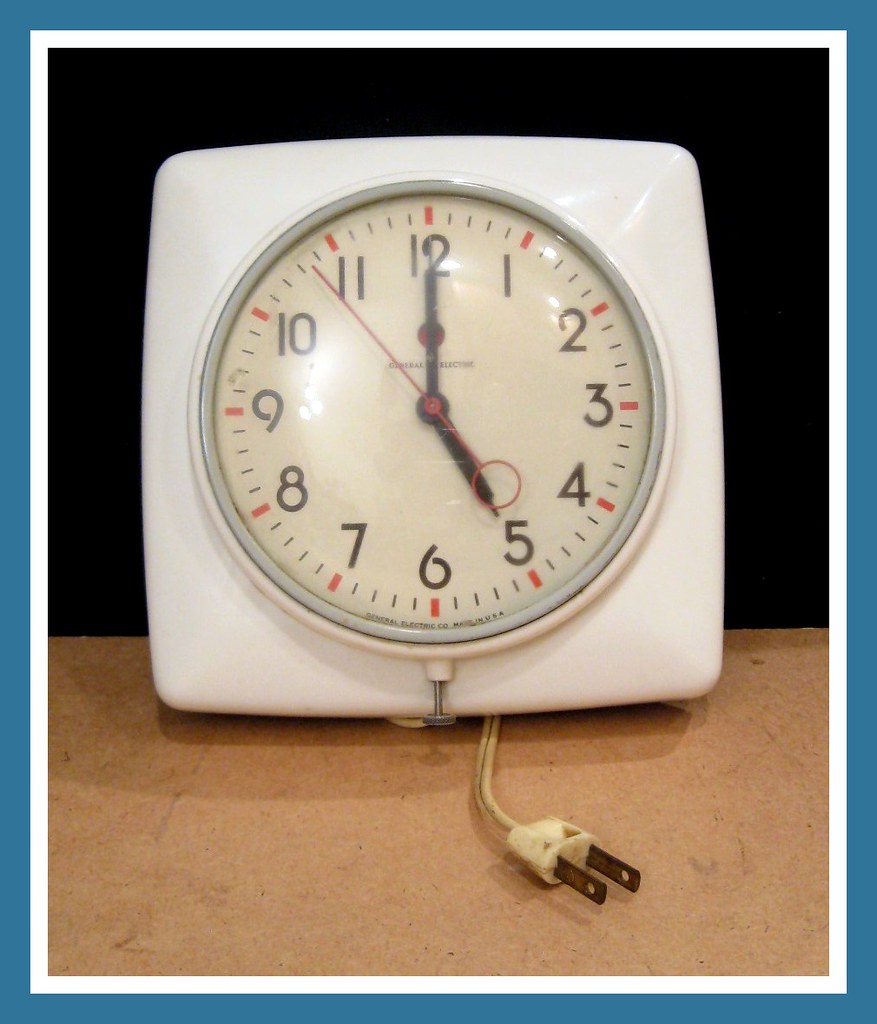The image depicts a vintage plug-in clock with a square white base, resting on a light brown tabletop. The clock has a circular face with black numerals ranging from 12 to 12, and features black hour and minute hands. The hour hand points to 5, while the minute hand points to 12. The red seconds hand is positioned just before the 11. Each numeral is marked by red dashed lines on the clock face, which has a black background. A white power cord extends from the bottom of the clock, with an old, white plug and brown prongs.